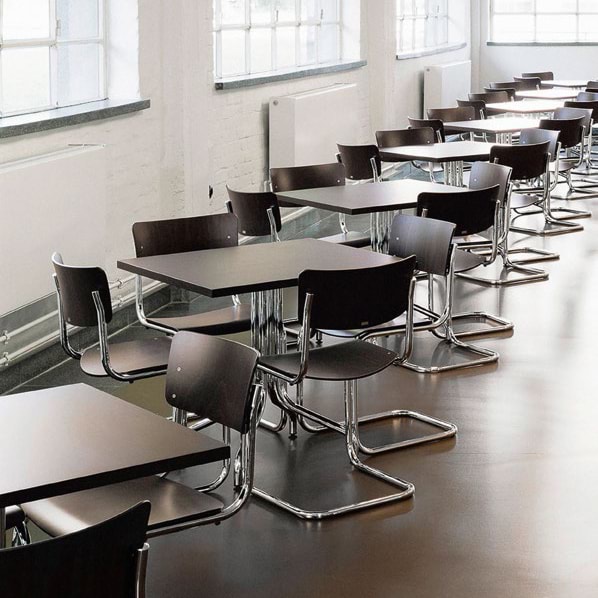The image depicts an institutional cafeteria with a meticulously organized layout. Square tables with chrome legs are each paired with four chairs, featuring a hardwood back and seat atop a curved chrome base. Large paned windows made of see-through blocks allow light to flood the stark, whitewashed room, which has bare walls save for a few white boxes mounted on them. Below each window are mantles that appear to be either granite or marble, and beneath the mantles are radiant heaters connected to visible pipes, likely carrying steam or water. The floor is a brownish concrete, contributing to the austere atmosphere of the space. The identical arrangement of tables and chairs—with no variation in their appearance—reinforces the impression of a highly regulated environment, possibly reminiscent of a hospital or mental health facility.